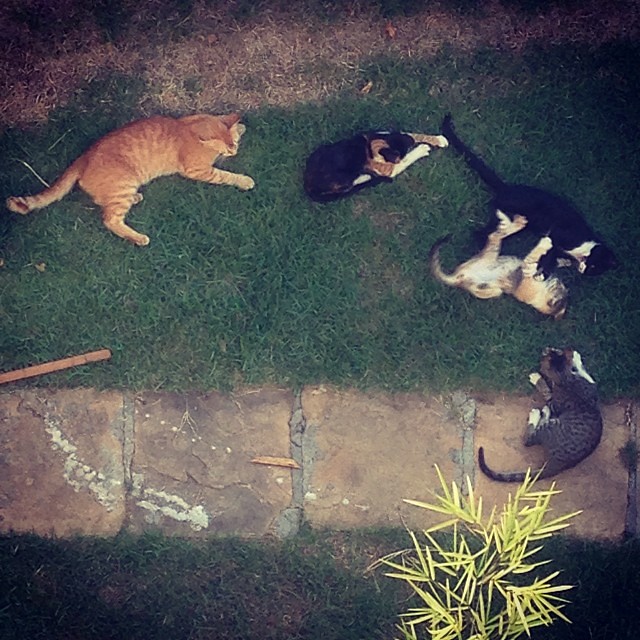The aerial image showcases a vibrant yard teeming with life, highlighted by five distinct cats. At the top of the image, an orange cat lies comfortably on a lush expanse of grass, facing the other felines. Adjacent to it on the left is a calico cat, while a tuxedo cat (black and white) and another calico display playful antics, rolling around joyfully in the center. A brown cat sits at the bottom, seemingly ready to join the fun. The bottom of the image features a wide stone pathway with sizable stones interlaced with white grouting, contrasting the green surroundings. To the bottom right, a small tree with long, spiky lime-green leaves adds a touch of nature's wildness to the serene setting.